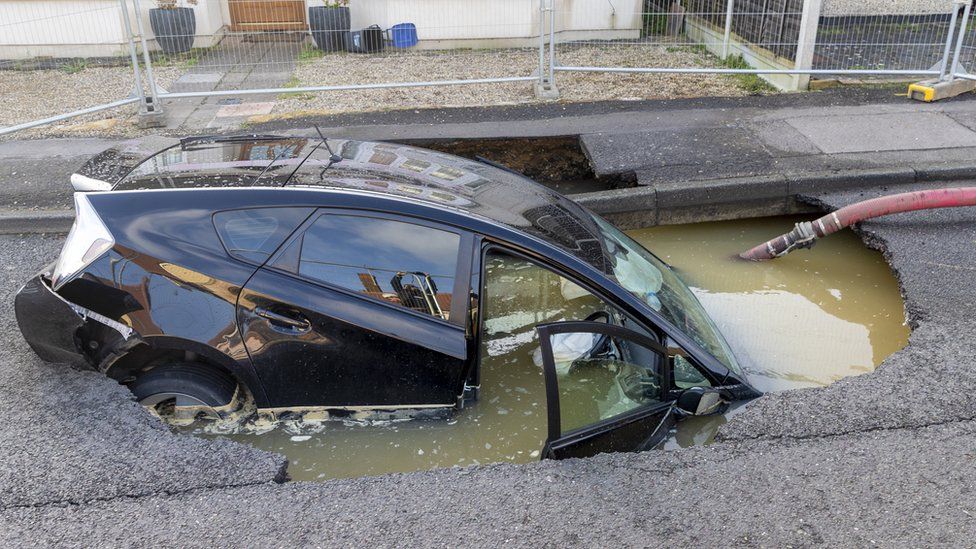In the image, a black Toyota Prius has fallen headfirst into a large sinkhole, completely submerging its front end and partially submerging the rear. The passenger door is ajar, revealing that the car's interior is filled with water. A sizeable red hose is actively pumping water out of the sinkhole. This incident has occurred on a collapsed roadway situated in front of a white house with a brown door. The house is bordered by a gated area adorned with some pots and stones, rather than grass. The image clearly shows that the car's steering wheel is on the right-hand side, suggesting the scene is set in a European country. Additionally, either the airbag has deployed or some internal car contents are floating inside. The street and surroundings appear chaotic, underscoring the severity of the sinkhole and the subsequent damage.